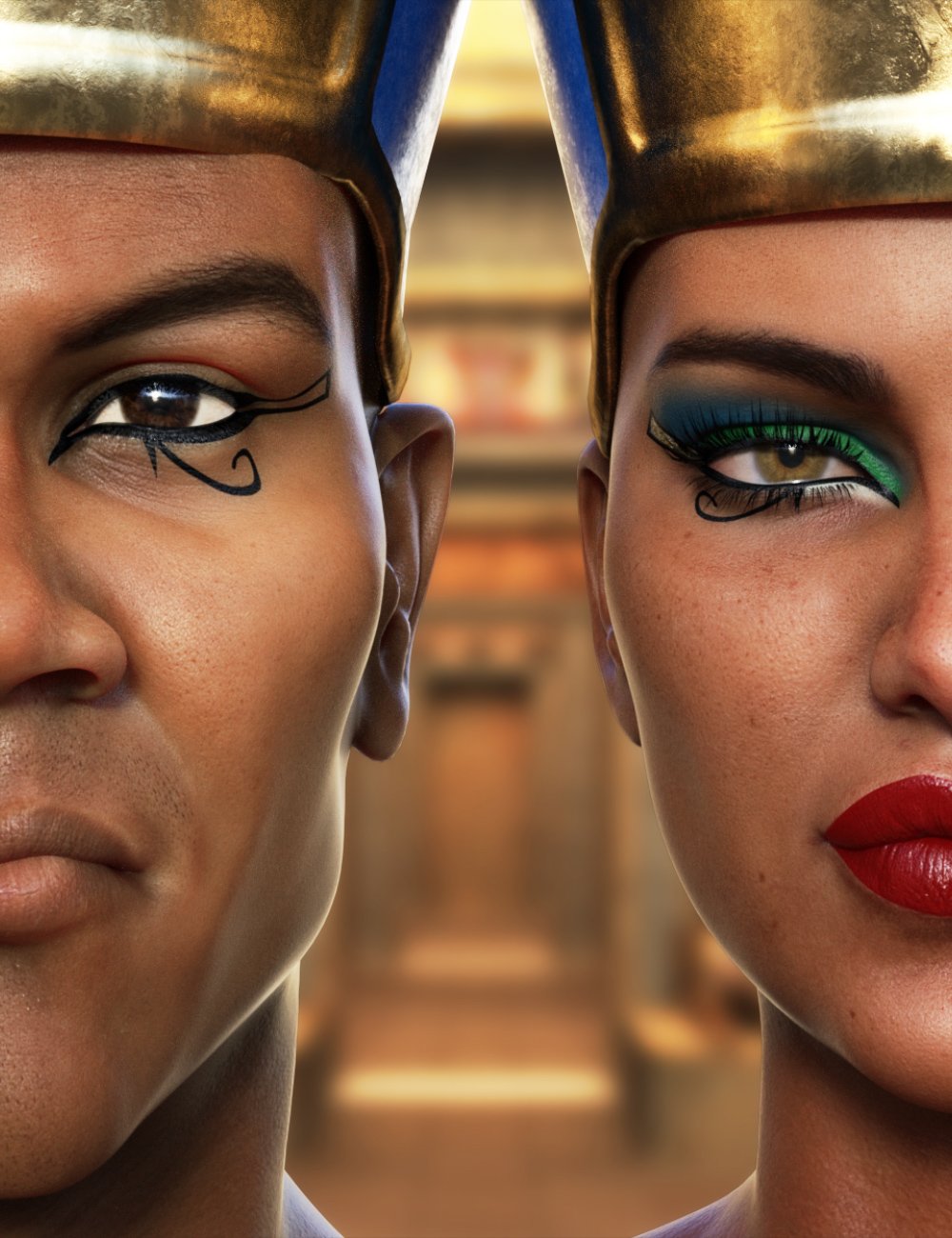The image portrays a digitally created, vertically rectangular scene focusing on the left halves of the faces of an Egyptian king and queen. Standing closely together, the king is positioned on the left with dark skin and strong cheekbones, adorned with a golden crown with blue accents. He has black eyeliner and eye pencil, akin to the eye of Horus, under his eye extending outward with a hieroglyphic mark. The queen, on the right, also has dark skin and is embellished with bluish-green eyeshadow, black eyeliner, and vibrant red lipstick. She sports a similar golden crown with blue accents and a hieroglyphic tattoo under her eye. The blurred background features an ancient Egyptian architectural style, including a vaguely visible palace door, reinforcing the royal and historic ambiance of the scene.